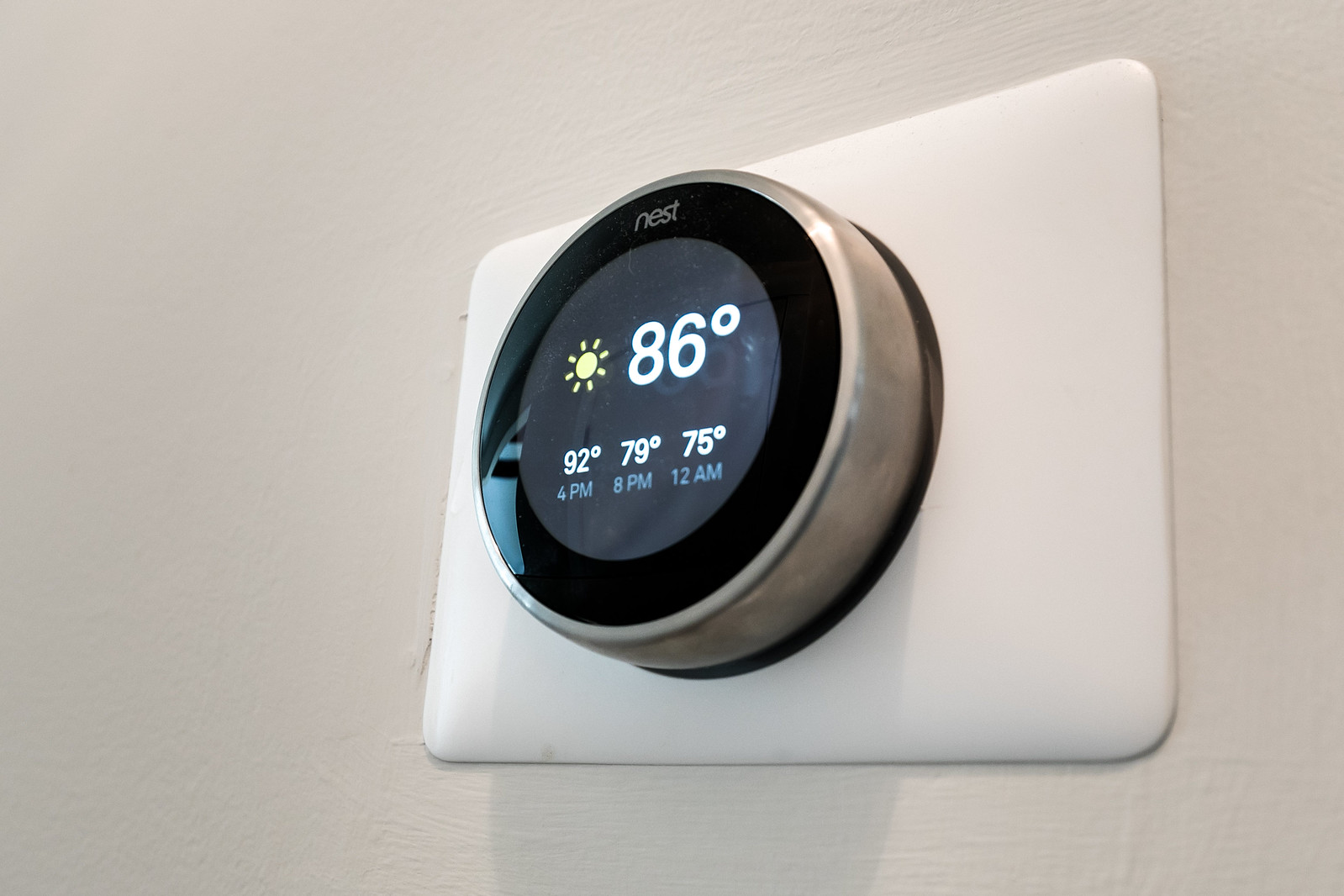In the image, we see a sleek, modern wall with a prominently featured device from the brand Nest. This device, known for its advanced thermostat capabilities, is designed to manage and regulate your home's air conditioning system. Even when you're not at home, you can program and control the temperature via a computer.

The main focus is a circular thermostat, approximately six inches in diameter, displaying various digital readouts on its screen. The display border is black, and at the center, it features a bright yellow Sun icon, which indicates the current weather condition. Directly below the icon, the temperature reads 86 degrees Fahrenheit, all presented in bold white digits for clarity.

Further down the screen, in slightly smaller yet still bold white text, the thermostat lists forecasted temperatures: 92 degrees at 4 p.m., 79 degrees at 8 p.m., and 75 degrees at 12 a.m. This detailed information is all housed within a clean, white frame reminiscent of a standard outlet cover, adding a touch of minimalist design to the device's high-tech functionality.